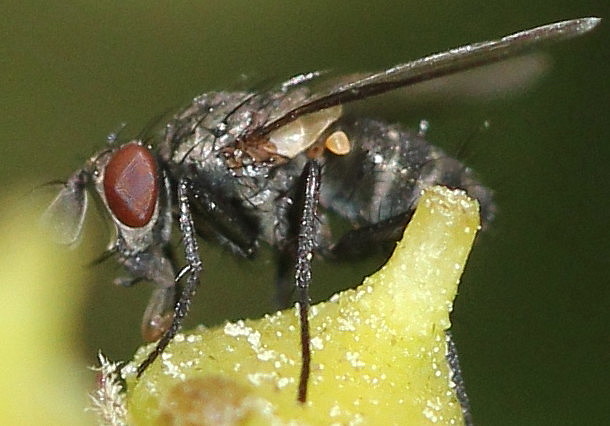This image is a close-up shot of a black insect, likely a fly, characterized by large red eyes. The fly is perched on a yellowish-green plant, which is dusted with what appears to be white pollen. The insect's translucent wings exhibit a slight brownish tint with a hint of silver. Notable features include its thin, hairy legs, partially extended wings, and prominent antennae or mouthparts, possibly mandibles, interacting with the plant. The background is entirely blurred, drawing focus to the textured details on the fly and the pollen-covered plant. The bottom left corner displays what seems to be a thumbprint, indicating a potential mishap during the photographing process. Overall, the image's zoomed-in nature captures the intricate details of the fly and its interaction with its environment, despite the slight blurriness.